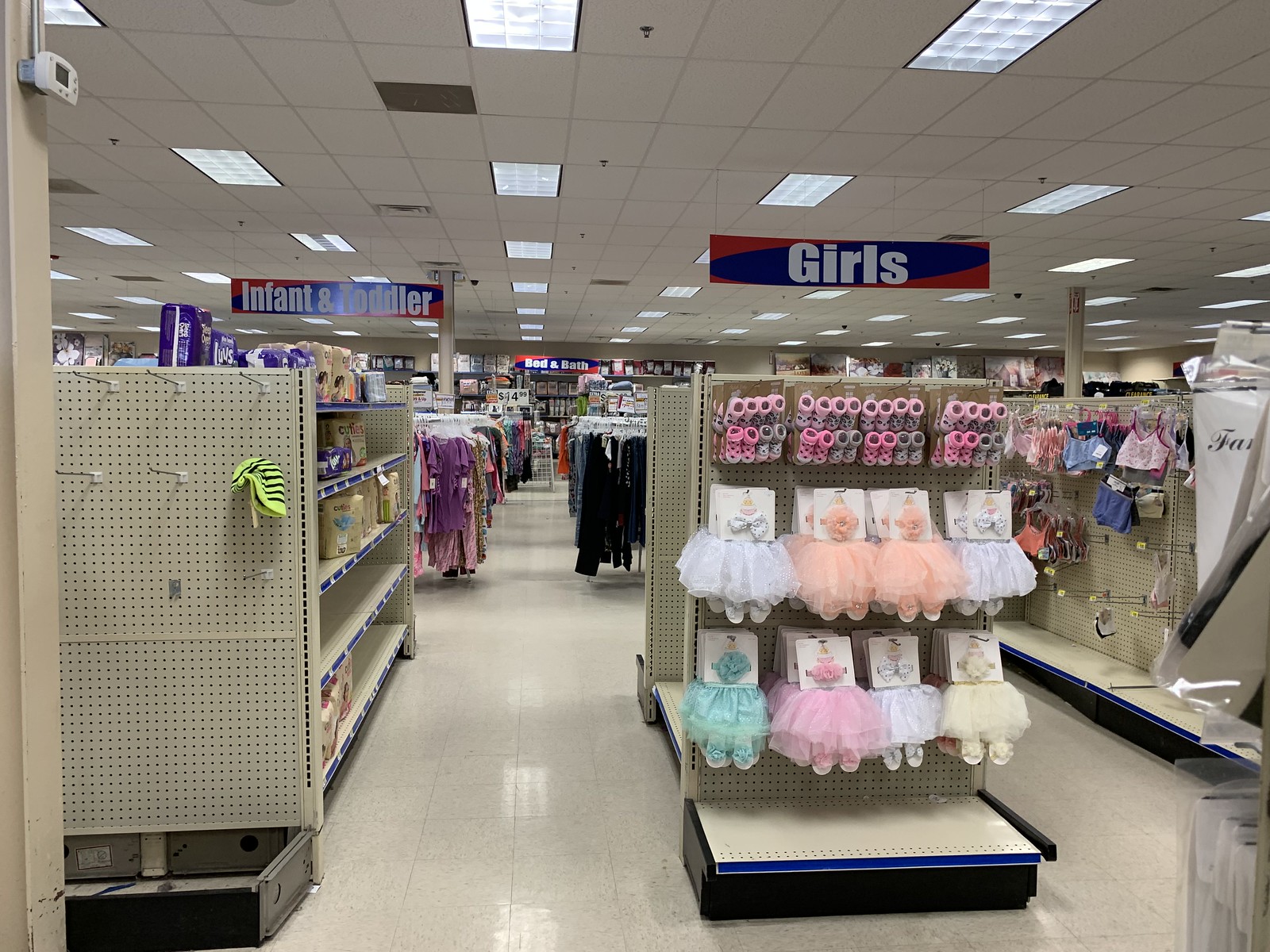In this photograph taken inside a retail store, the focus is on a display rack located in the girls' section, clearly marked by a sign that reads "Girls" in bold red and blue text with white letters. The top row of the display features an array of tiny toddler shoes, meticulously organized in pairs. Beneath the shoes, several racks are adorned with colorful ballerina tutus, complete with matching accessories, evoking a whimsical and playful atmosphere. Adjacent to these items are additional metal shelves stocked with various infant and toddler essentials. In the background, the store extends into more racks filled with an assortment of clothing. A sign on the far wall indicates the "Bed and Bath" section, suggesting a well-organized store layout. The ceiling is lined with typical office fluorescent lighting, casting a bright, uniform light over the entire scene.